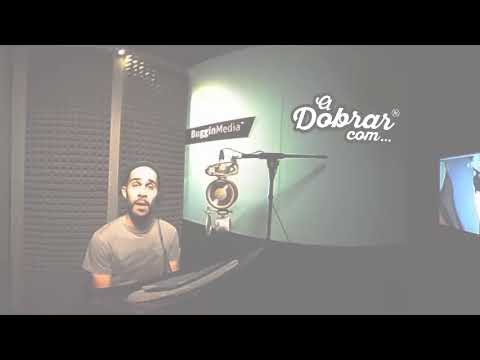In this grainy, fisheye-lens photograph, a man with a dark skin tone and short black hair sits in a radio booth-like room, facing the camera. He is visible from the chest up, appearing to be seated at a desk that is in shadow. The man, who has a beard and mustache, wears an olive green t-shirt and seems to be engaged in speaking into a fancy metallic-style cardioid microphone positioned in front of him on the desk. A black cable suggests he likely has headphones on. The image has a grayed-out, hazy overlay, making the room appear oversaturated and brighter than it might be in reality. To his left is a dimpled, soundproof foam wall, while the rest of the wall features a sage green color. On the far right of the image, near the edge, a small cropped television screen is visible. Text is partially legible on the wall beside the screen, with fragments like "Doorbar," "adobar.com," and "media" faintly discernible in the hazy, muted backdrop.